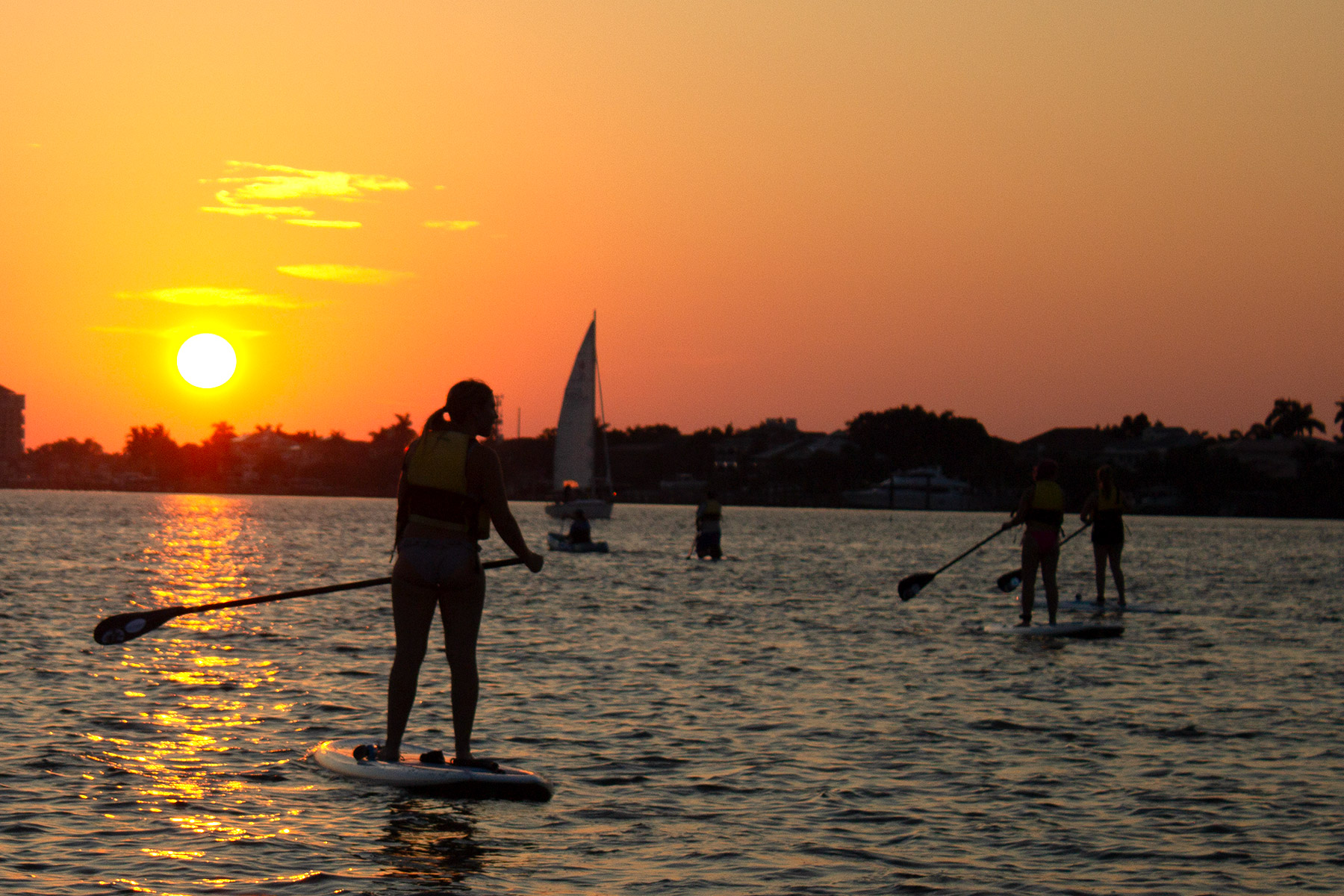In this vibrant evening scene, several people are engaging in stand-up paddleboarding on a serene body of water, which could be a lake, river, or a calm stretch of the ocean. The water presents gentle waves and an enchanting blue hue. Notably, a woman with a ponytail is prominently positioned in the foreground; she stands confidently on her white paddleboard, holding her paddle to the left. To her right, two more individuals are visible on their own paddleboards, all donned in yellow life vests that catch the fading light. In the backdrop, a sailboat drifts lazily, adding to the tranquil atmosphere of the setting. The sunset paints the sky in glorious shades of orange, red, and brilliant yellow, with the round sun sitting low on the horizon. This colorful spectacle casts a warm glow over the water, causing it to shimmer with reflections of the sunset. The horizon is defined by a shoreline dotted with trees, including palm trees and other varieties. Some boats are moored along this shore, with houses peeking through the foliage. The overall scene captures a moment of peaceful recreation under a beautifully illuminated sky, with the paddlers leisurely enjoying their time on the water.